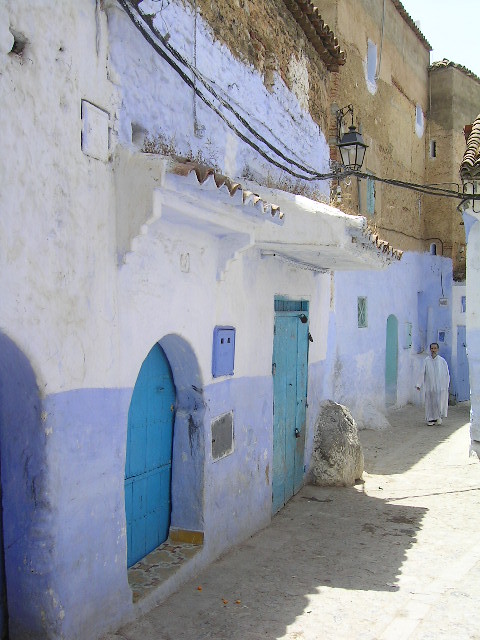This photograph captures a charming cobblestone alleyway that is reminiscent of a Mediterranean or Greek village. The narrow street is lined with interconnected stone buildings, featuring a blend of traditional beige, brown, and gray hues. The exterior of these buildings showcases a striking mix of white and blue, with fresh white paint dominating the upper sections and light blue or periwinkle accents adorning the lower portions and doors. 

Flanking the alley on the left, blue doors and decorative shelves—some of which hold non-flowering, brownish plants—lend a quaint, picturesque charm. The scene is illuminated by bright sunlight, casting distinct shadows across the area, and delicate wires overhead hint at lighting fixtures not currently in use. 

A figure in white—wearing a robe and matching shoes, with short dark brown hair—walks towards the viewer from the right side of the image, drawing the eye to the center. Further details emerge such as a blue vent with black holes, indents in the lower walls, and a yellow tiled step near the first door on the left. Above the doors, small white awnings provide subtle shade, while the rooftops display a mix of black, brown, and natural stone colors. Finally, a touch of the cloudy sky peeks through the upper right corner, completing this idyllic and detailed scene.